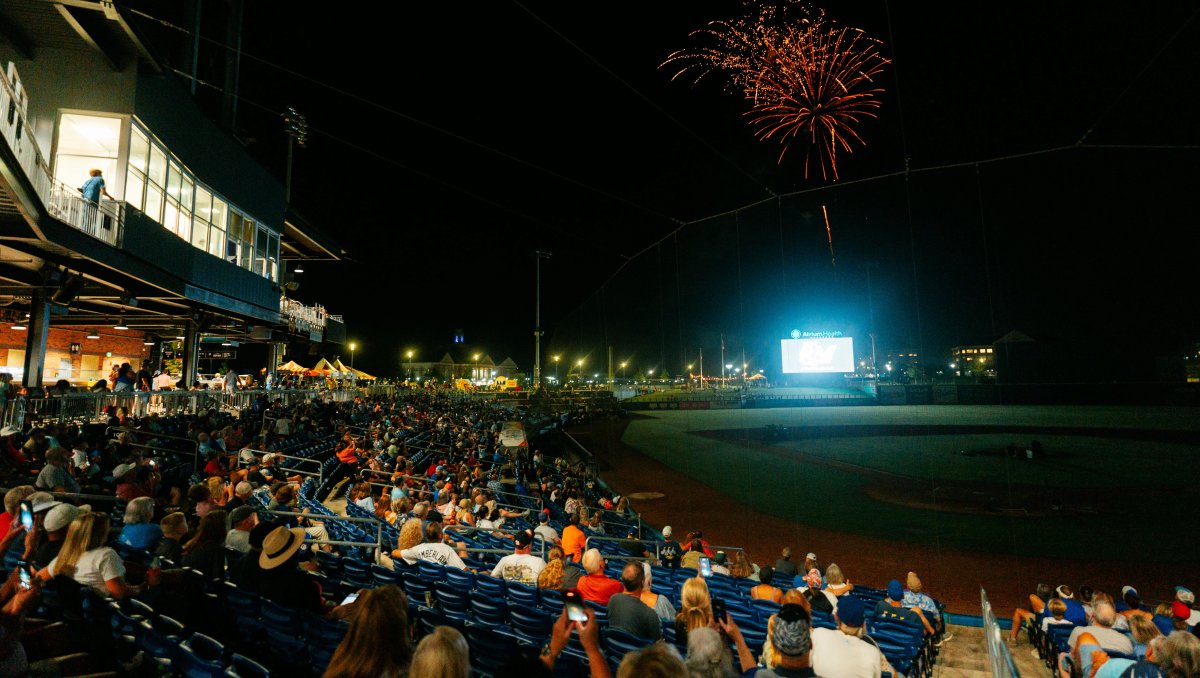The nighttime photograph captures a lively scene inside a minor league baseball stadium. The sky is pitch black, sharply contrasting with the brilliantly lit grandstand and a vivid white jumbotron brightening the outfield. Blue seats run around the stadium, with spectators dispersed throughout, some leaning over the railing. The green grass at the center highlights the open-air atmosphere of the venue. Above, a spectacular firework display lights up the sky with a plume of red and orange-yellow bursts. Numerous fans hold up their phones, capturing the dazzling fireworks against the dark backdrop of the sky.